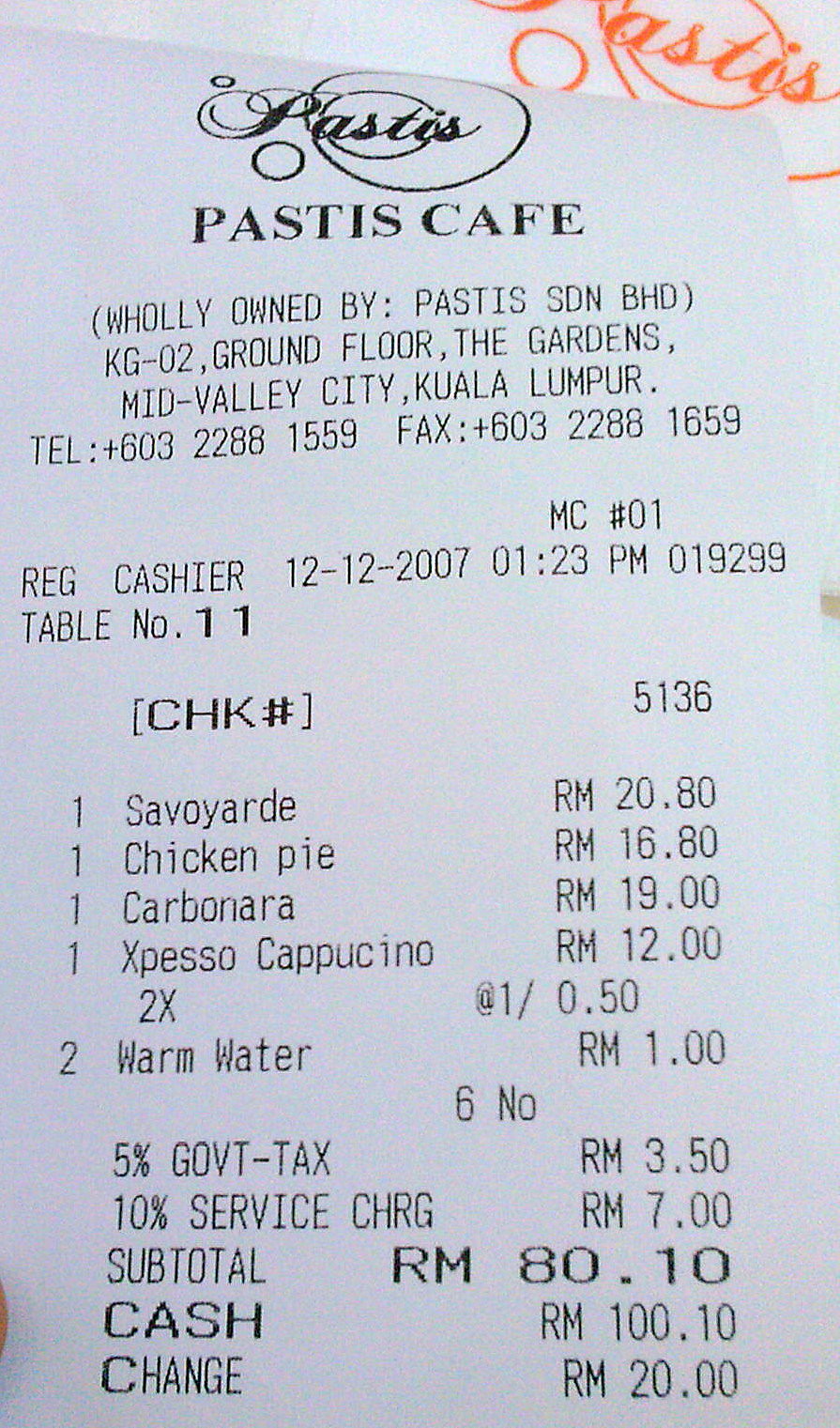A high-resolution photograph of a receipt from Pasties Cafe, prominently featuring an orange logo adorned with decorative font and circular accents on the right-hand side. This same logo is repeated at the top of the receipt, clearly identifying the venue as Pasties Cafe, a business wholly owned by Pasties SDN Ph.D. The cafe is located on the ground floor of The Gardens in Mid Valley City, Kuala Lumpur. Contact information is provided, including a phone number (603-2288-1559) and a fax number. The receipt indicates that the purchase was made on December 12, 2007, with the customer seated at table number 11. The total amount paid for the transaction was $80.10.